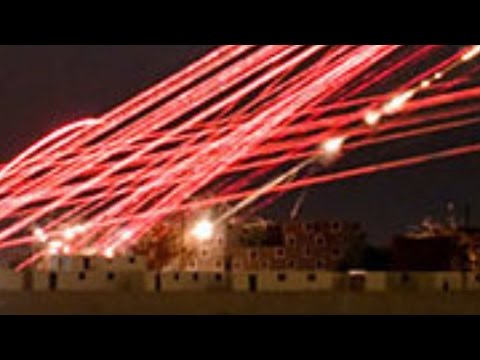A screenshot, likely from a movie or YouTube video, is characterized by cinematic black bars on the top and bottom of the image. The scene, set at night, reveals a dark sky. It captures a dramatic moment where numerous red laser beams are either penetrating into or emanating from a house. These lasers vary in shades from light pink to dark red, creating a striking contrast against the darkness. The intensity and variety of the red hues add a sense of urgency and tension to the scene, enhancing the overall dramatic effect of the nighttime setting.